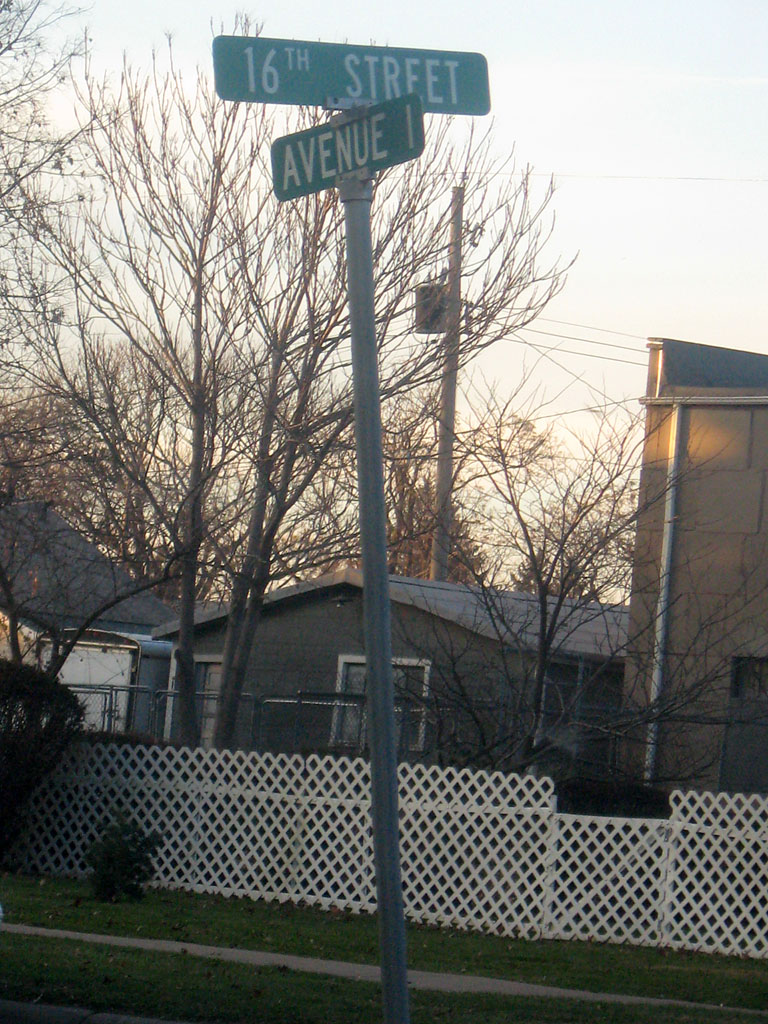In this serene late afternoon scene, a street sign marks the intersection of 16th Street and Avenue 1 in a residential neighborhood. The signs are positioned in a crisscross manner, clearly indicating the directions of the streets. The setting sun casts a warm, golden light, creating a picturesque glow on the houses and the area around. A portion of the sidewalk is visible, bordered on either side by lush green grass and a few verdant bushes. Adjacent to the street sign stands a white lattice fence, adding a charming touch to the scene. In the background, there are two prominent houses. One is a modest gray house, while the other, on the right, resembles an industrial structure with its brown concrete façade and white gutters running down the sides. Metal fences by these buildings lend an additional layer of texture to this tranquil snapshot of suburban life.